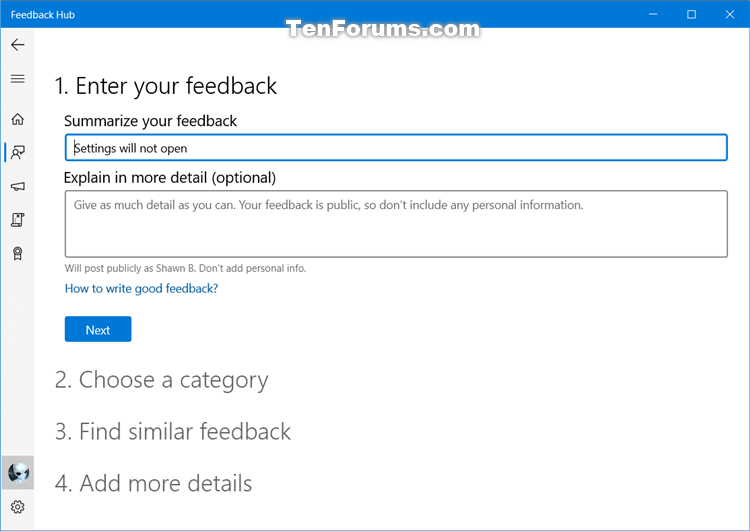At the top of the image, there's a prominent blue banner with the text "Feedback Hub." To the right of this banner, there is a horizontal line intersected by a small box and an 'X' icon, which are partially overlaid on the blue banner. Below this, in a white box with a gray halo effect, the text "10forms.com" is displayed.

On the left-hand side of the image, a vertical gray index is visible. This index features a series of icons stacked from top to bottom: an arrow pointing left, three horizontally stacked lines, a house icon, a person with a speech bubble, a megaphone, a map, and a ribbon. At the very bottom left, there is a horizontal gray bar containing a globe icon and a gear symbol.

In the main white content area of the image, text begins with "1. Enter your feedback." Following this is the prompt "Summarize your feedback." Underneath this prompt, there is a large blue outlined rectangular box with text indicating "settings will not open." The next line reads "Explain in more detail (optional)." Below this, a large gray outlined rectangular box advises, "Give as much detail as you can. Your feedback is public, so don't include any personal information."